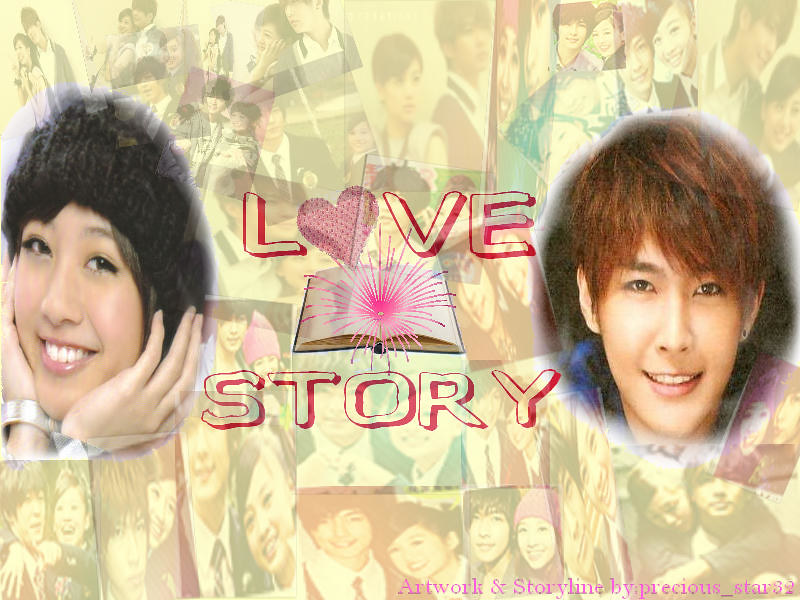This detailed and cleaned-up caption incorporates elements from all three descriptions:

The image showcases a fan-made artwork titled "Love Story" by PreciousStar32, featuring two young Asian figures—a male and a female—against a collage backdrop of their various life moments. The female, positioned on the left, has smooth skin, short black hair, and is wearing a winter beanie. She is smiling gently, revealing shiny white teeth and wearing pale red lipstick. Her chin is cupped in her hands adorned with a shiny, flat bracelet on her right wrist. On the right, the male figure has short, reddish hair styled in a pixie cut, dark eyes, and a similar open-mouth smile. Between them, in the center, bold yellow letters outlined in red spell out "L heart V E," with a heart shaped like a pink sprout dotted with red symbolizing "Love." Below it, the words "story" complete the phrase "Love Story." The bottom right corner features the inscription "Artwork and storyline by precious_stars" in pink lettering. The background is a hazy blend of images portraying the duo in different poses, possibly representing their journey together through various stages of life.